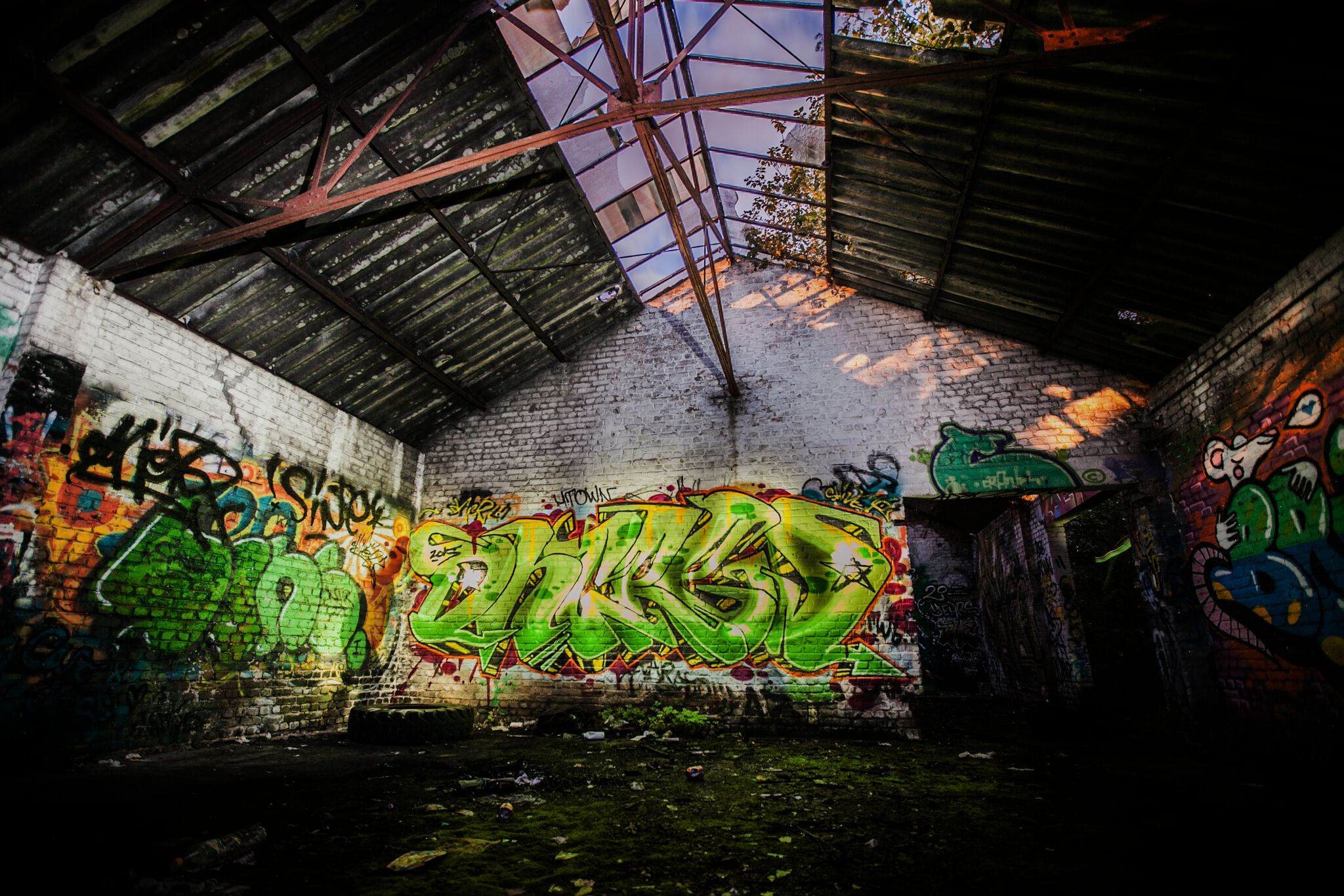The image depicts the interior of an abandoned structure, likely an old greenhouse, showing signs of decay and artistic vandalism. The building is constructed from gray or white brick and has a distinctive roof with windows that once allowed sunlight to stream in, some of which are missing or broken. Copper beams support the ceiling, adding to the industrial aesthetic. Graffiti covers the walls extensively, with prominent green, lime green, orange, yellow, and red hues creating an intricate layer of urban art. The left wall features vibrant graffiti with multiple colors, while the right wall showcases a detailed depiction of a rat holding green letters and surrounded by a speech bubble with a heart. The back wall also displays various graffiti, blending words and images. The ground is littered with debris, including some trash and a tire, contributing to the dilapidated atmosphere. Two dark doorways lead to other parts of the building, shrouded in shadows and mystery.